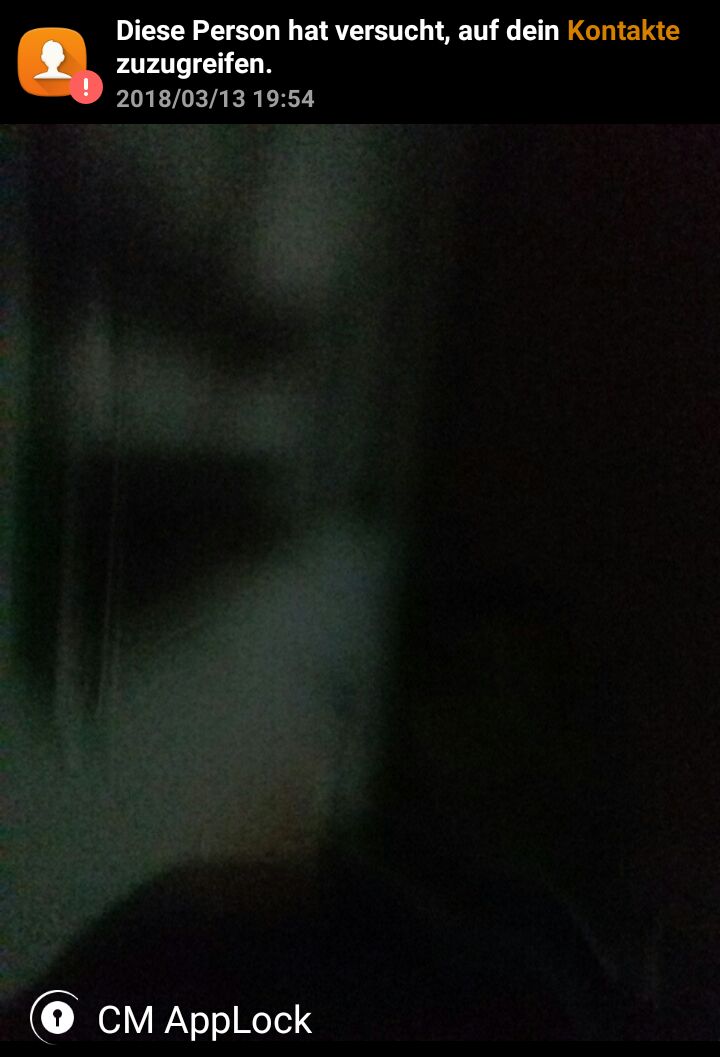The image predominantly features text. In the top left corner, there is a square icon with an orange background. Within the square, a white illustration of a person's head and shoulders is depicted. Adjacent to this icon, on the bottom right, is a circular element with a pink background housing a white exclamation mark. To the right of these graphical elements, text is displayed.